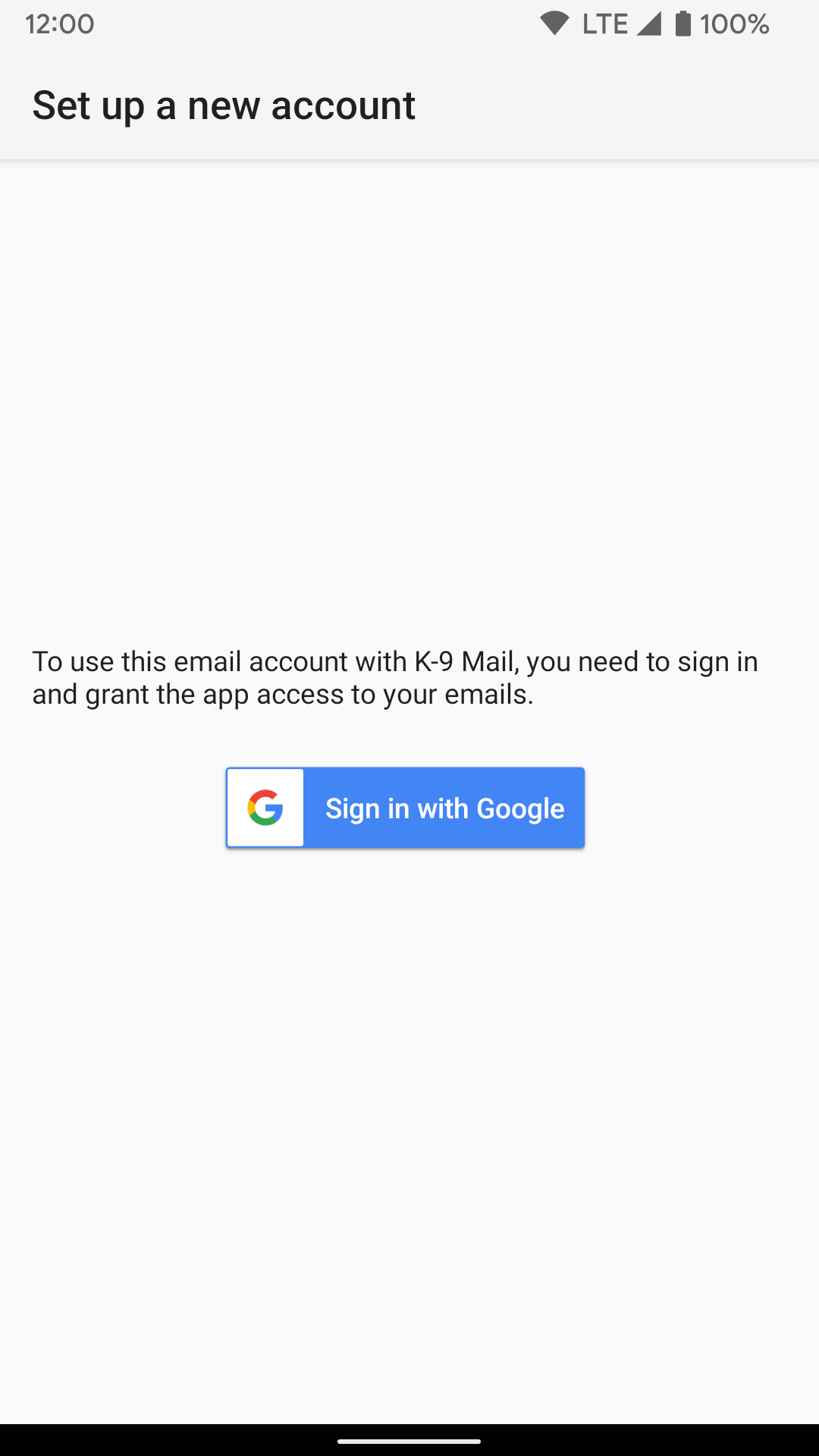This screenshot, taken in portrait mode from a phone, displays the interface for setting up a new email account in the K-9 Mail app. In the upper left-hand corner, the time is shown as 12:00, while the upper right-hand corner indicates a full battery charge at 100% and an LTE network connection. 

Dominating the top portion of the screen, bold text instructs the user to "Set up a new account" against a gray background. Below this message, centered on the screen, there is a prompt stating, "To use this email account with K-9 Mail, you need to sign in and grant the app access to your emails." Directly beneath this instruction is a prominent, light blue button that reads "Sign in with Google." To the left of this button is the Google logo.

The background remains a uniform gray until the very bottom of the screen, where a black bar extends from the bottom left to the bottom right. Centrally located within this black bar is a thin white line. This minimalistic interface clearly guides the user towards signing in with a Google account to proceed with setting up their email in the K-9 Mail app.